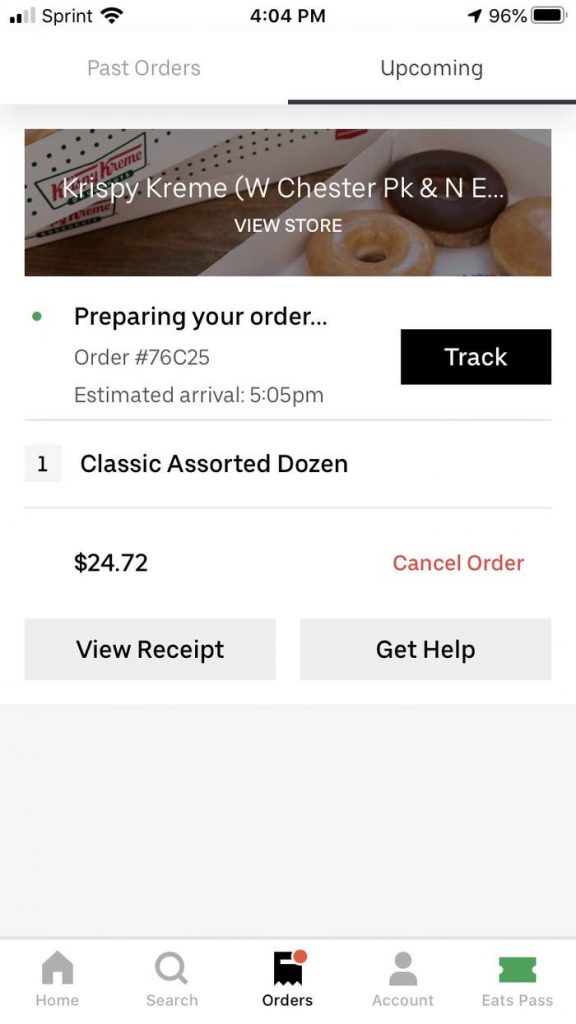The image depicts a smartphone screen displaying an order summary from a food delivery app. 

In the top left corner, there are icons indicating the phone's signal bars, the carrier (Sprint), and Wi-Fi signal. The current time is shown in the center as 4:04 PM, and the battery level on the right shows 96%.

Below this status bar, the screen is divided into sections. The first section contains two tabs: "Past Orders" and "Upcoming Orders," with "Upcoming Orders" underlined, indicating it's the active tab.

The next section shows details of an active order. "Krispy Kreme (West Chester PK and NE...)" is the store name, followed by a "View Store" link underneath. Below this, an image of a box of Krispy Kreme doughnuts is displayed, albeit partially obstructed by the text overlay.

The text overlay indicates that the order is currently being prepared, with an order number of 76C25. The estimated arrival time is 5:05 PM. A black button labeled "Track" with white font allows the user to track the order.

Details of the order show a classic assorted dozen doughnuts priced at $24.72. Under this, there is a red button for canceling the order, a gray "View Receipt" button, and another gray button labeled "Get Help."

At the bottom of the screen, there is a navigation bar with icons for "Home," "Search," "Orders," "Account," and "Eat Pass." The "Orders" icon has a red circle indicating a notification and is highlighted in black, while the other icons are grey, except for "Eat Pass," which has a green icon but grey text.

The total cost of the order is mentioned to be $25.